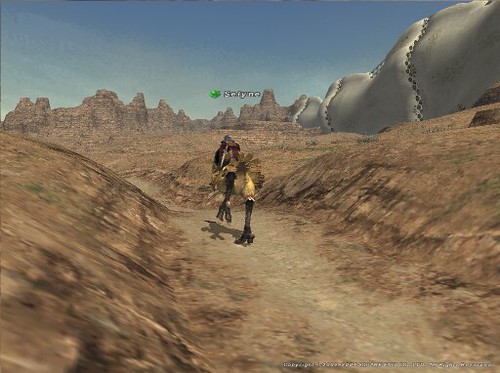The image appears to be a screenshot from a video game, possibly resembling the style of "The Legend of Zelda." The central focus is a character riding a large, ostrich-like bird, which is primarily yellow with a brown fan-shaped tail. The bird's powerful back legs are clearly visible as it traverses a barren desert landscape devoid of plants or trees. In the background, a distant mountain range is visible, adding depth to the scorched and desolate environment. To the right, there is a peculiar gray structure, potentially a rock formation, featuring what look like hand and footholds. The sky above is a vivid blue with few, if any, clouds, contributing to the arid atmosphere of the scene.